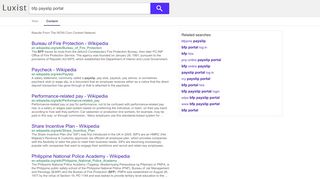A screenshot of a webpage is displayed, with the website name "Luxist" prominently shown in the top-left corner in clear, readable text. Directly to the right of the website name is a search bar, identifiable by the magnifying glass icon within it. The rest of the text on the image is too small and blurry to be decipherable. The image contains no photographic elements and no presence of people, animals, plants, buildings, vehicles, or any other discernible objects. The screenshot focuses solely on the website's header area, emphasizing the Luxist branding.